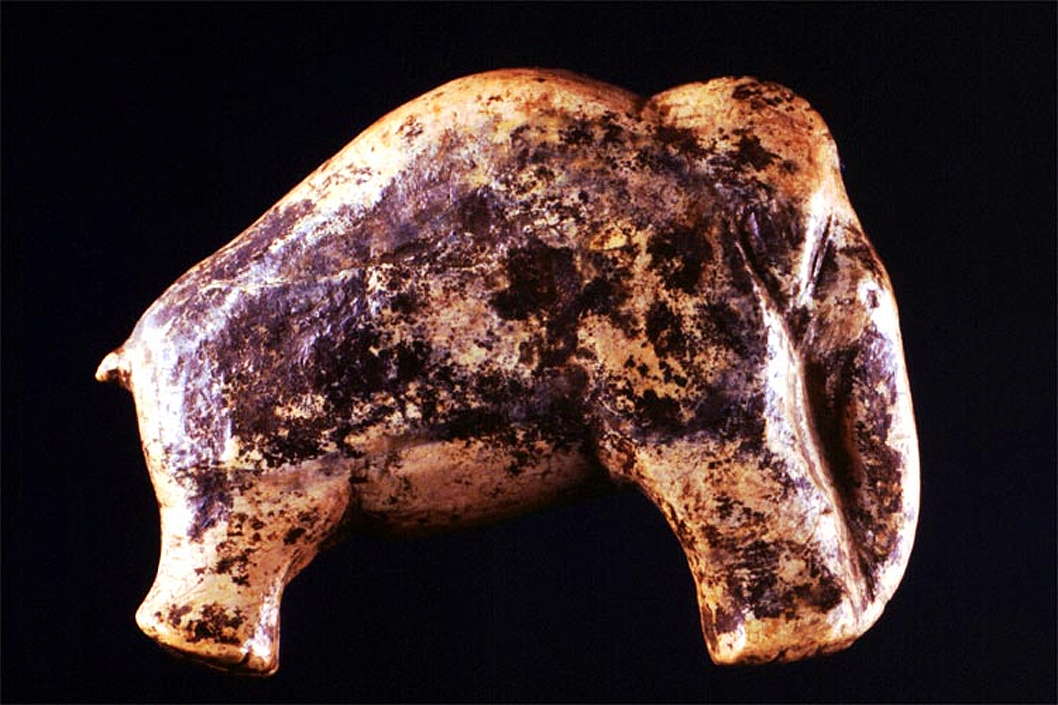The image showcases an ancient artifact crafted in the shape of an elephant, presented against a jet-black background that makes the object stand out prominently. The artifact, viewed in profile, reveals only the two right legs, a small tail, and the head with a downward-facing trunk. It appears to have been carved from either wood, ceramic, or another hard material. The original surface seems to have been a tan or sandy brown, now heavily worn and discolored with large black blotches and spots, indicative of significant aging and weathering. The sculpture lacks visible details such as eyes, which may have either faded or never been present. The object’s overall condition suggests a long history, adding to its sense of antiquity.